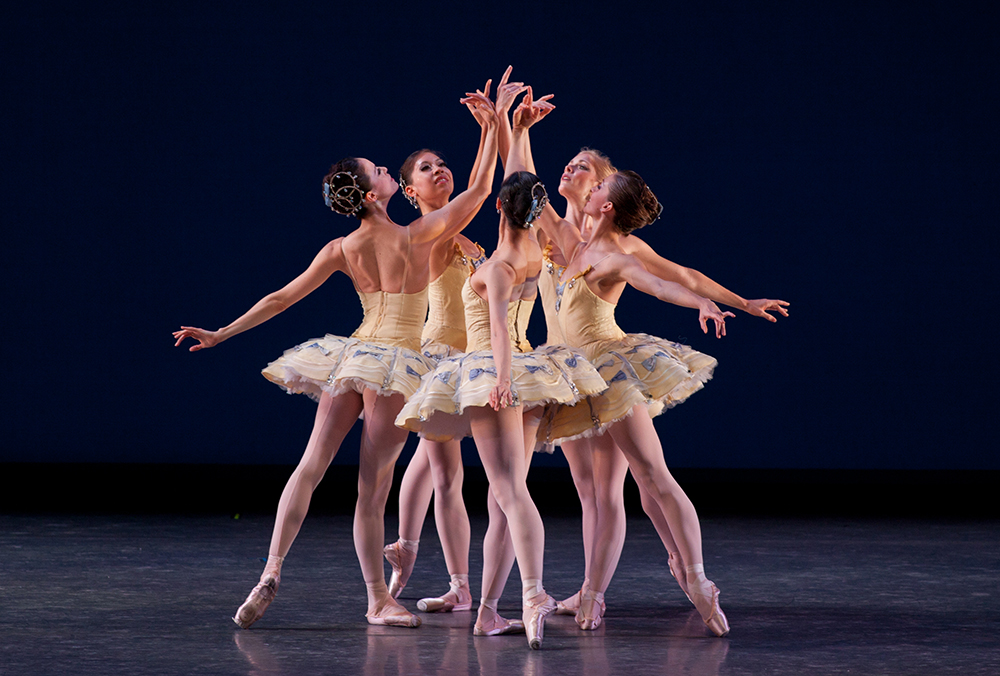The image features a group of five female ballet dancers performing on a stage with a black marble floor and a dark blue-to-black gradient background. Each dancer is dressed in a custard yellow tutu adorned with a striking butterfly wing pattern in black and yellow at the bottom of the dress. They wear pink ballet shoes and ballet tights that complement their outfits. The dancers are positioned in a circular choreography, their hands raised and touching in the center, creating an elegant and unified pose. Their hair is styled neatly with gold and blue hairpieces pinned at the back, adding a touch of sparkle to their appearance. The dancers' graceful movements and coordinated attire give the performance a vivid and captivating quality.